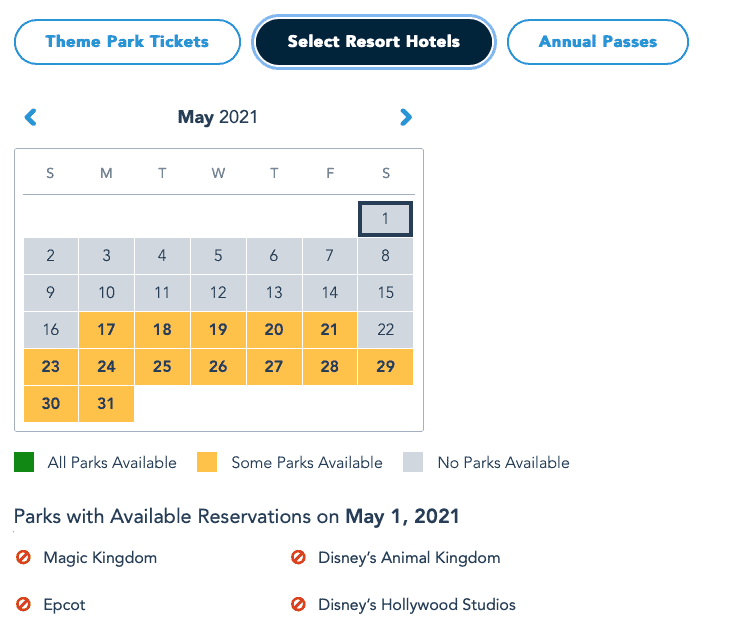This screenshot, taken from a webpage, appears to originate from a Disney theme park's booking system, potentially for Magic Kingdom or Epcot. At the top of the webpage, there are three clickable tabs: "Theme Park Tickets" on the left, "Select Resort Hotels" in the middle, and "Annual Passes" on the right. The "Theme Park Tickets" and "Annual Passes" tabs are displayed in white with blue lettering, indicating they are not currently active. The "Select Resort Hotels" tab is active, as signified by its black background with white text.

Directly below the tabs, a calendar for May 2021 is prominently displayed. Navigation arrows, colored blue, are present on either side of the month label, allowing the user to move to previous or subsequent months—though the narrator implies moving back would be unnecessary. Below the month label, individual dates are shown. Specific days are boxed to indicate availability: May 1st is marked with a black box and the text "some parks available," while other dates such as the 17th to 21st, 23rd to 29th, and 30th to 31st are also shown as available during the month. Dates before the 17th are noted as having no parks available, highlighting limited availability within the selected time frame.